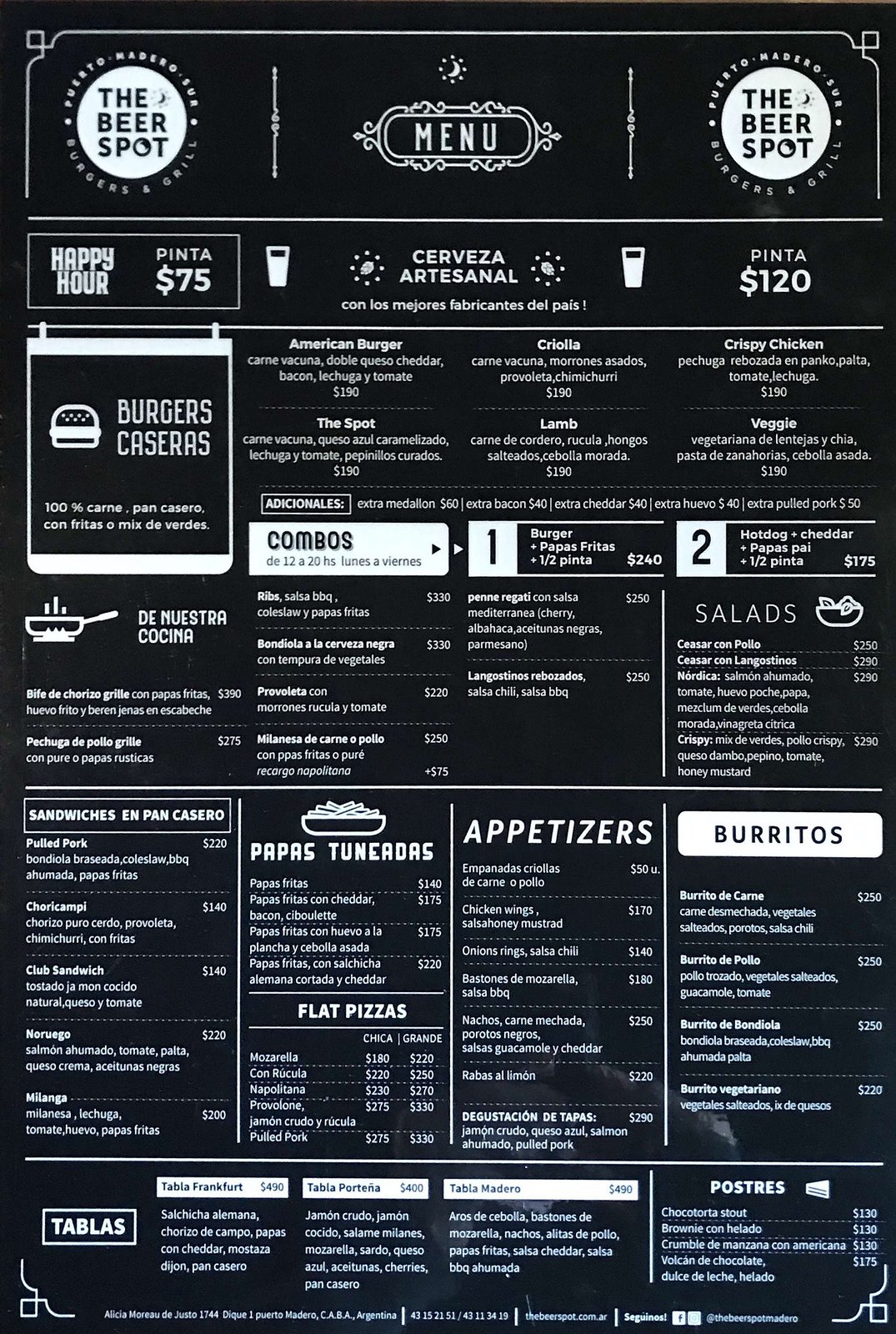The image features a detailed, colored menu with a sleek black background and crisp white text, providing a striking contrast for readability. Positioned at the top left and right corners are prominent white circles containing the restaurant's name, "The Beer Spot." Centrally, the menu displays the word "Menu" and the enticing heading "Happy Hour."

Highlighted offerings include:
- Pinta for $75
- Cerveza Artisanal for $120.

Underneath, a section dedicated to burgers lists several tempting varieties:
- American Burger
- The Spot
- Crayola
- Lamb
- Crispy Chicken
- Veggie.

The menu also features a "Combos" section, with most of the items described in Spanish:
- Combo #1: a burger, fries, and half of a pint.
- Combo #2: a hot dog with cheddar cheese, half a pint, and "papas" (potato dish).

Additionally, the menu includes categories for:
- Sandwiches
- Potato Dishes
- Appetizers
- Burritos.

Despite some of the text being too small to read clearly, the menu meticulously outlines a variety of enticing options, catering to diverse tastes and preferences, albeit predominantly in Spanish.